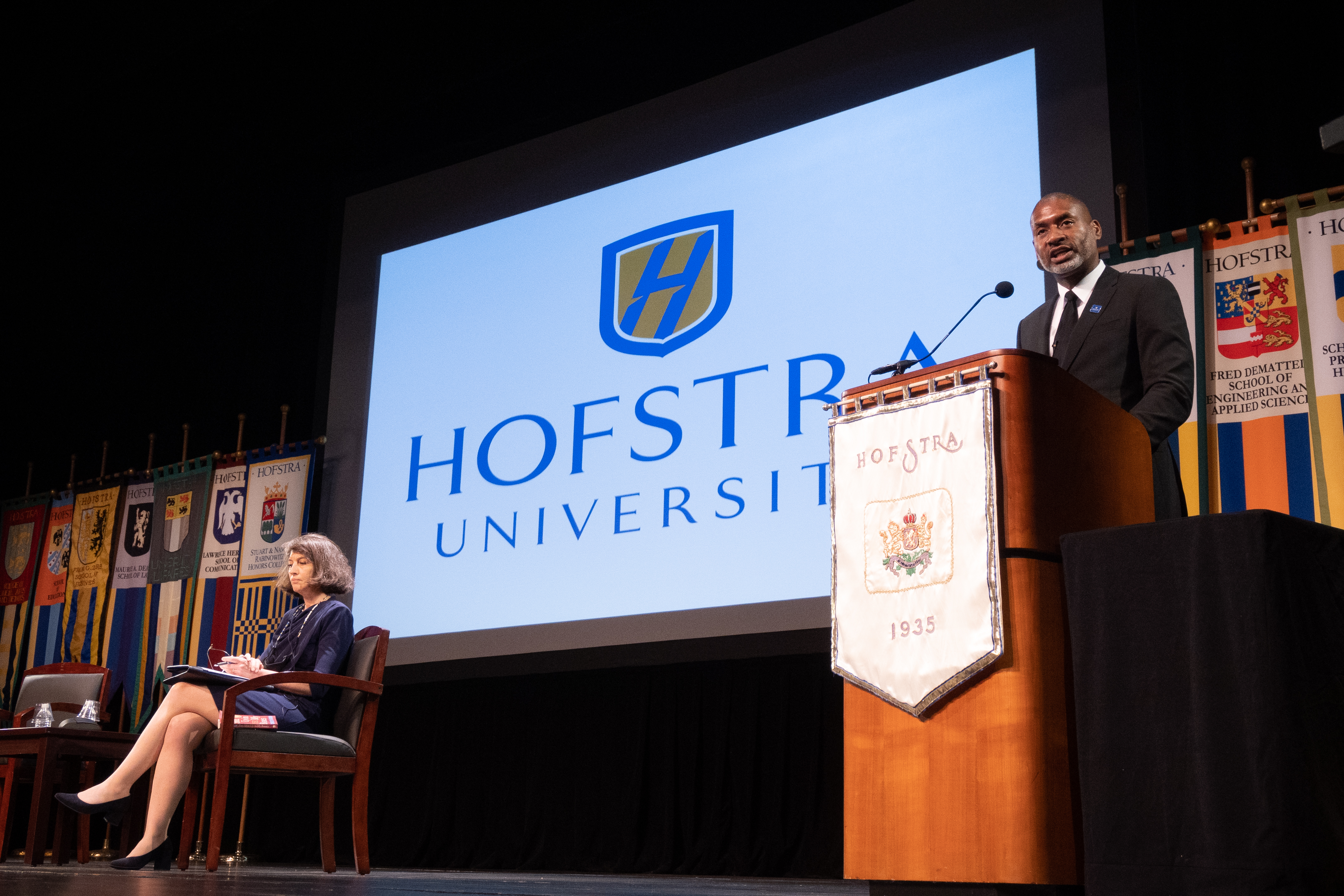The color photograph captures a speaking event at Hofstra University, viewed from the perspective of an audience member near the stage. Central to the image is a large display screen prominently featuring the Hofstra University logo. The stage setup includes various banners, with one in front of the podium emblazoned with the Hofstra shield and the year "1935."

On the right side of the stage, a middle-aged African-American man stands behind a podium. He is wearing a dark suit with a white dress shirt and his mouth is open, indicating he is addressing the audience. The man has a shaved head.

To the left of the screen, a woman with medium-length brown hair, who may be Caucasian, Asian, or Latina, is seated on a wooden chair with leather backing. She is dressed in a navy blue jacket and skirt, holding a folder on her lap, and has a contemplative expression as she looks out into the audience. The scene suggests a formal and engaging atmosphere at a university event.